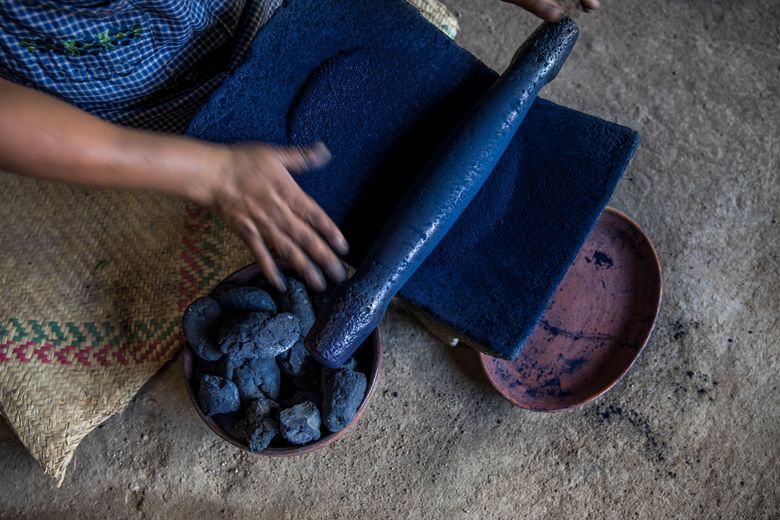The image captures a close-up scene of an artisan engrossed in a meticulous craft, seated upon a straw mat, possibly on a stone surface. The artisan, whose hands are the only visible part, is engaged in rolling out a long, cylindrical rod covered in a vibrant cobalt blue dye over a rectangular mat also saturated with the same blue hue. To the artisan's right, there is a bowl filled with small blue rocks or similarly textured material, and in front of the mat lies an empty oval bowl showing traces of blue residue. The individual's hands appear slightly stained by the dye, indicating immersive participation in the process. The person is either wearing a shirt or a blue dress, suggesting traditional attire, and their actions seem to hold cultural significance, as inferred from the careful handling of the materials involved.